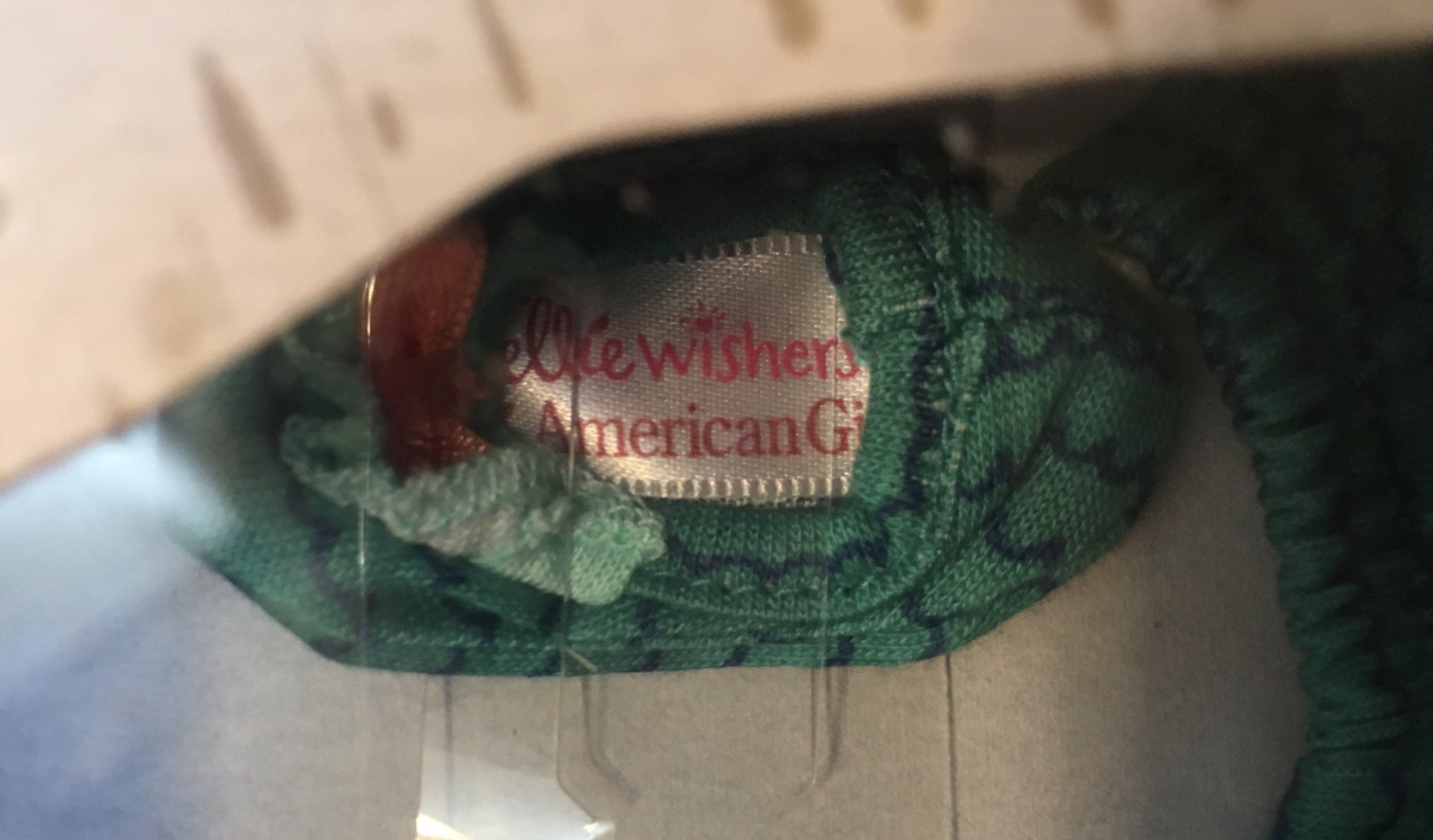Here's a detailed caption for the image:

"A detailed close-up of a fabric tag attached to a piece of clothing, possibly a shirt, blouse, or dress, laid out on a white background. The garment itself is made of green fabric adorned with intricate dark blue patterns and lines. The tag, which is centered in the image, is white and displays red text partially readable as '...wishes American...,' with some of the text obscured or cut off. White threads are seen hanging loosely from the tag, indicating it might be newly sewn or coming undone. Below the tag, there is a glimpse of another white fabric layer, likely the inner lining of the garment."